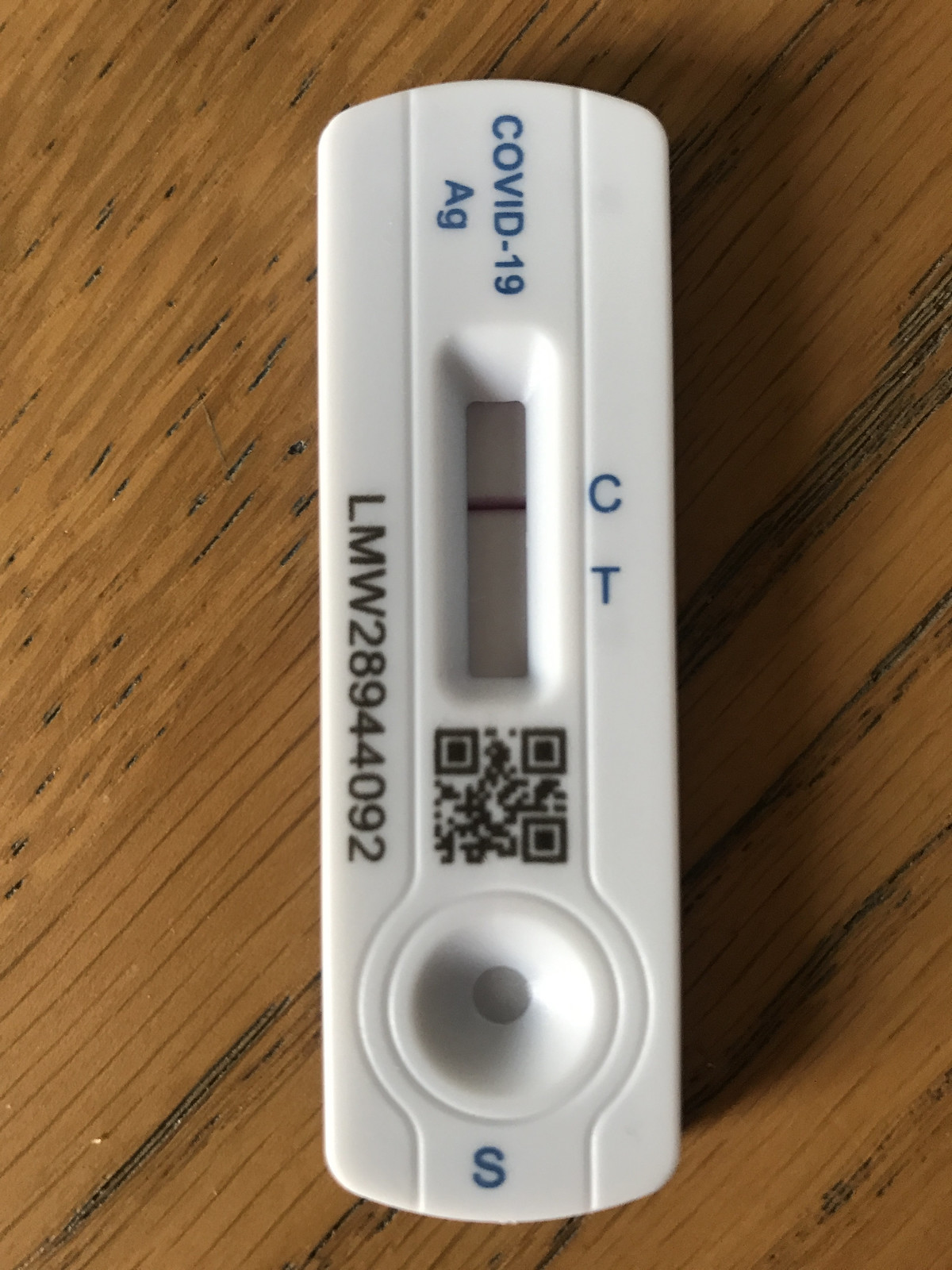A white plastic COVID-19 test lies on a bright brown wooden table, its rich grain clearly visible. The test, shaped like a rectangle with rounded corners, features a complex design. Running along the side of the test is the imprint "LMW 289 44092." Adjacent to this, there's an area demarcated with a rectangle and a circle. Within the rectangle, a red line points towards the label "C," aligned with another label marked "T." The phrase "COVID-19 AG" is inscribed next to the rectangle, while a black and white QR code occupies the space to its right. Further to the right, inside the circle, a smaller circle and a tiny indented spot denote the drop application area, labeled underneath with an "S."